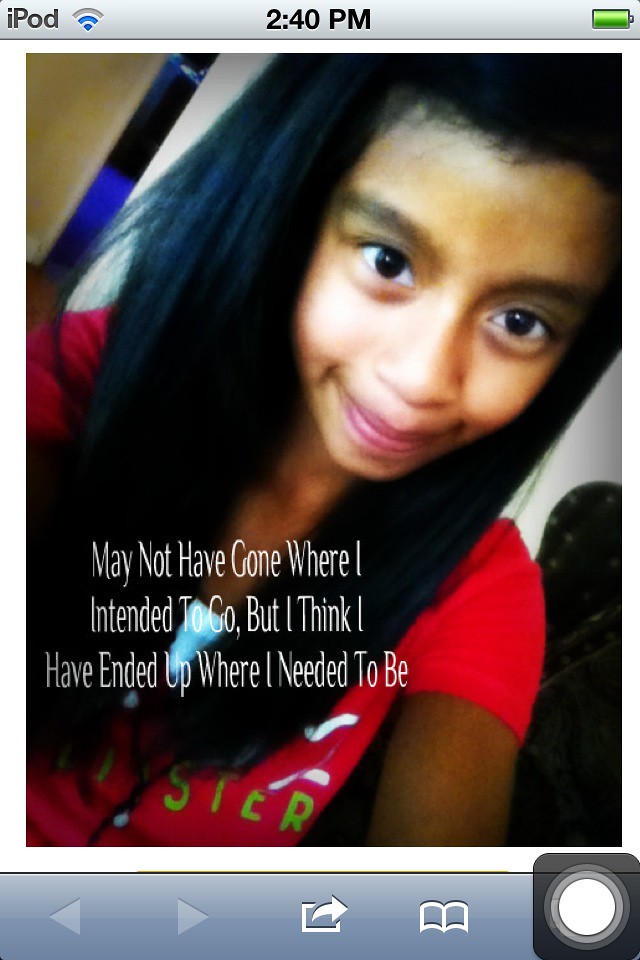This image appears to be a screenshot from an iPod interface. The top of the screen displays the text "iPod" accompanied by a Wi-Fi signal icon showing two out of three bars. This is followed by the current time, "2:40 PM," centered at the top, and a battery symbol at the top right indicating a full, green battery.

Dominating the screen is a photograph of a girl who appears to be Hispanic with black hair, brown skin, and brown eyes. She is smiling and wearing a pink Hollister shirt, although her hair slightly obscures the shirt's logo. Superimposed on the image is a quote in white text: "May not have gone where I intended to go, but I think I have ended up where I need to be."

Below the image are navigation and function buttons. Greyed-out left and right arrow keys flank a share button in the center. To the right of the share button is a bookmark button, and in the bottom right corner, there is a screen record button.